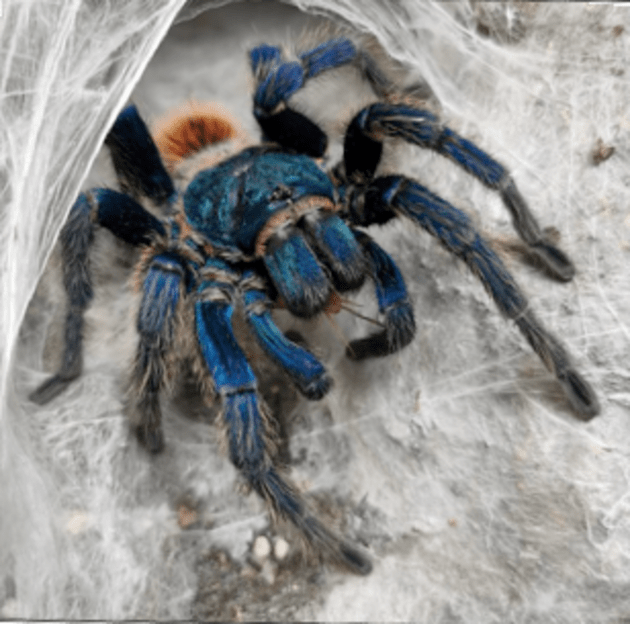This image captures a striking scene featuring a large, blue tarantula with black-tipped, hairy legs and a reddish-orange abdomen. The tarantula, which appears healthy, is positioned atop an expansive, sheet-like web that resembles a funnel. The intricate web spreads around what seems to be a natural surface, possibly a tree or the forest floor, with some dirt visible. The spider's head and legs are a vivid blue, transitioning to black at the tips, creating a stark contrast against the reddish-orange hue at the back. This detailed scene also shows the tarantula consuming a cricket it has caught, highlighting the spider's predatory nature within its meticulously constructed web habitat.